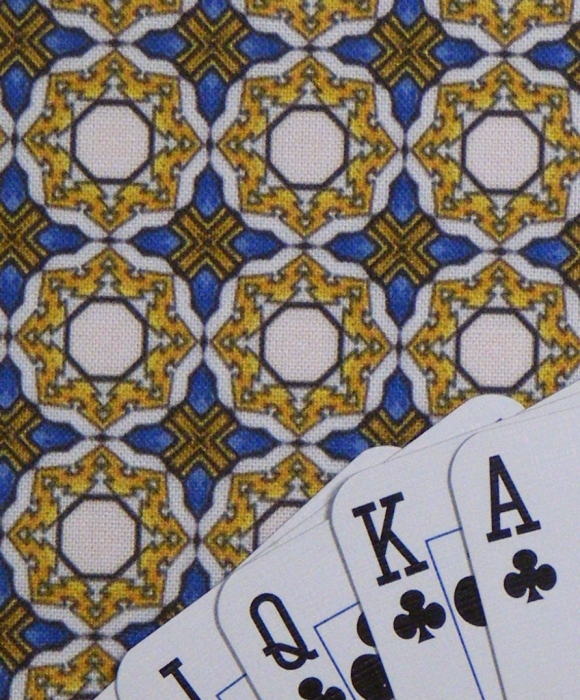In the image, there are four visible playing cards: the Jack of Spades, the Queen of Clubs, the King of Clubs, and the Ace of Clubs. Additionally, there's a fifth card, partially visible with just the corners shown. The background of the photo features a design reminiscent of stained glass windows often seen in churches. The intricate pattern includes colors such as white, yellow, blue, and black. The exact nature of the background is unclear, but it resembles fabric, possibly a tablecloth, with two distinct designs visible, one of which is partially in the shape of arcs or segments. The overall scene evokes a sense of elegance and intricate artistry.